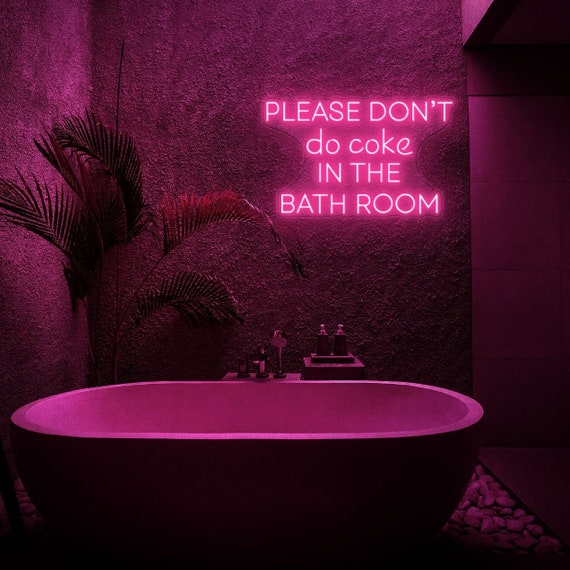This photograph of a bathroom reveals an eclectic and moody setting dominated by purple lighting that casts a vibrant hue across the entire space. The room, featuring high ceilings, is marked by a stark, rugged texture on its walls, reminiscent of coarse popcorn or rough concrete, giving it a distinctive character. Central to the scene is an elliptical, white bathtub, designed with a deep basin and positioned on a bed of medium-sized stone pebbles, adding a natural, spa-like element to the room.

Hovering above the tub is a neon sign that reads, "Please don't do coke in the bathroom," illuminated in bright pink-purple neon, adding a quirky and rebellious touch to the ambiance. To the left of the tub stands a palm plant, its green fronds interspersed with a few yellowing leaves, injecting a hint of freshness into the otherwise dark and enigmatic setting. Adjacent to the tub on a wooden pedestal sits an assortment of toiletries, including soap dispensers and lotion bottles, underscoring the room's functional aspect.

The exit from the bathroom appears to be to the right, where the rough-textured walls meet to form a corner, potentially leading out of this visually striking and thoughtfully decorated interior.